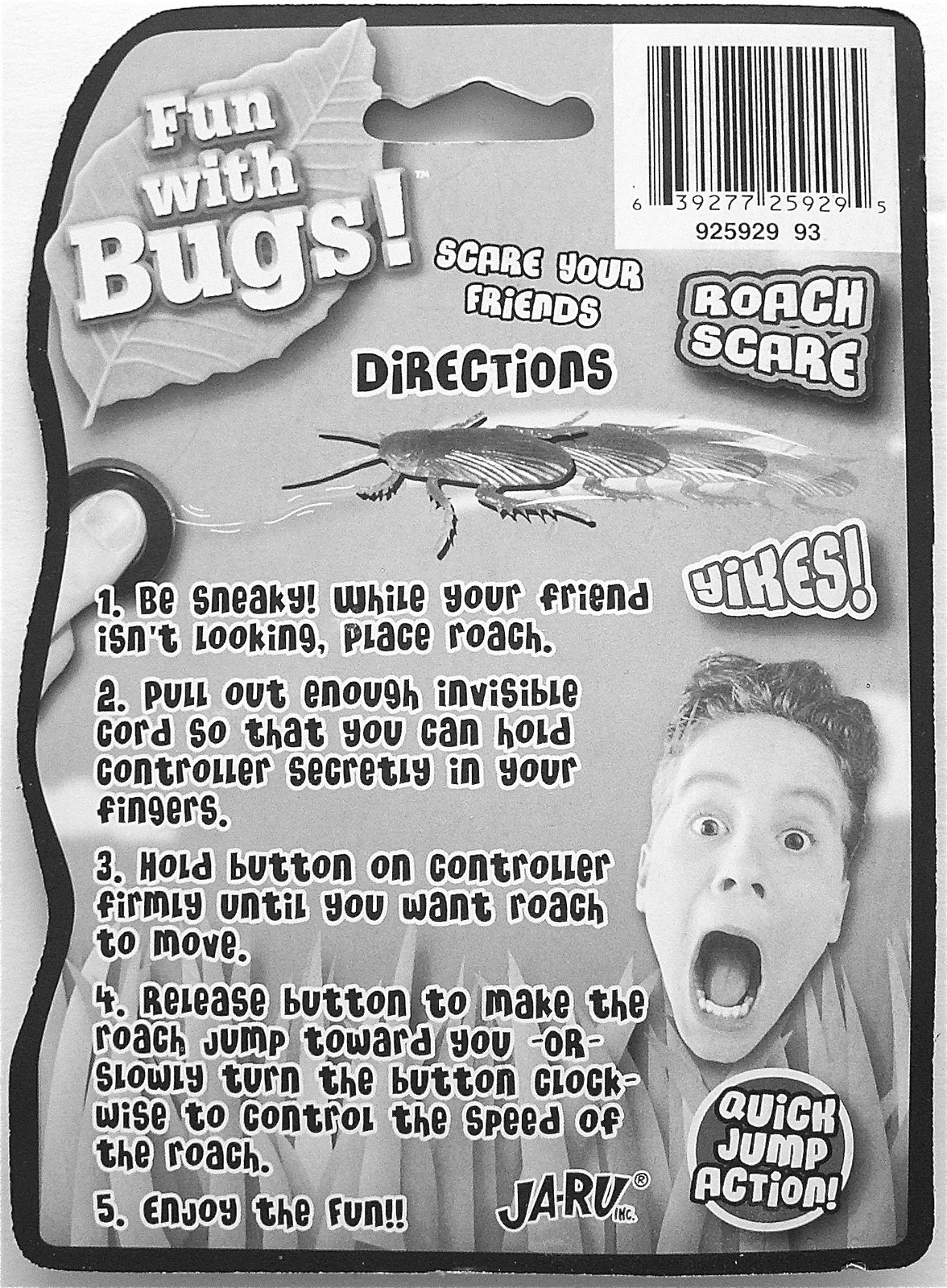The back of the toy packaging is presented in black and white and features a detailed layout. At the top, you can see the UPC code numbered 639277259295, with smaller text beneath reading 925929. To the left side, there's a heading in bold that says "Fun with Bugs." Adjacent to it on the right is an image of a leaf. Underneath, the text "Scare your friends" is displayed, followed closely by "Roach Scare" to the right.

Beneath this, you see the outlined directions for using the toy. A detailed illustration of a bug that resembles a cockroach accompanies these instructions. The step-by-step guidelines are as follows:

1. **Be sneaky** - While your friend isn't looking, place the roach in a concealed spot.
2. **Yikes** - Pull out a sufficient amount of invisible cord so that you can secretly control it with your fingers.
3. **Hidden Control** - Hold the button on the controller firmly until you want the roach to move.
4. **Roach Movement** - Release the button to make the roach jump toward you, or slowly turn the button clockwise to control the roach's speed.
5. **Enjoy the Fun** - Experience the thrill of surprising your friends.

Additionally, the packaging highlights "Jaru Quick Jump Reaction" and features an image of a child with a surprised expression, his mouth and eyes wide open to illustrate the excitement and reaction the toy aims to provoke.